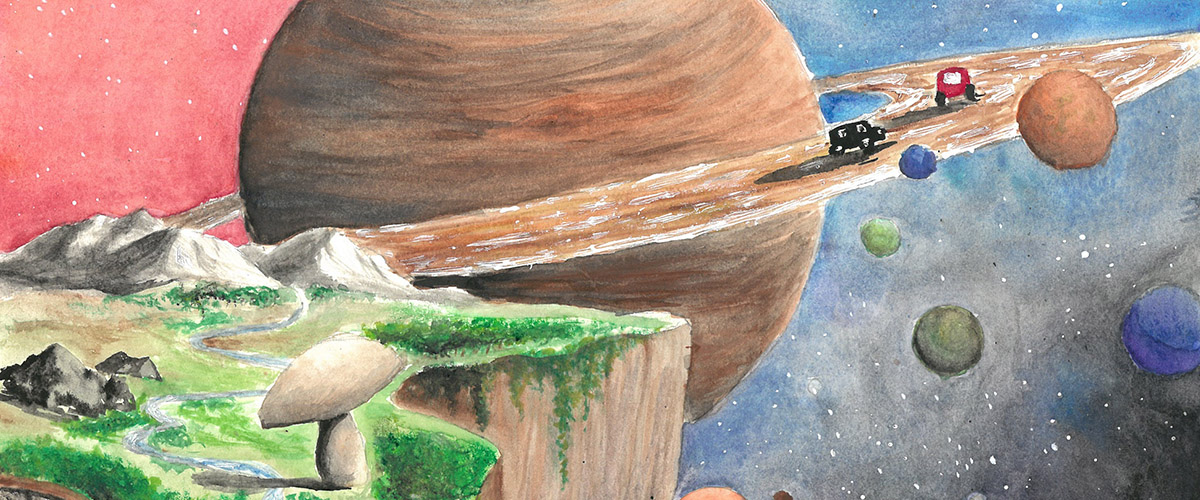The artwork is a sci-fi-inspired drawing, centered around the planet Saturn with a distinguishing ring. The ring resembles a winding road with two vehicles—one black with visible passengers and one red—driving on it. Surrounding the planetary rings are five floating moons: a large rusty-brown moon, a small blue moon near the black car, a light green moon slightly below, a darker green moon beneath the blue one, and an almost fully visible blue moon on the right edge of the image. 

In the foreground, a rocky cliff adorned with green foliage and moss runs down to the bottom of the image, with a white, mushroom-shaped structure on the front left. The backdrop of the scene transitions from a pink and blue sky on the right to an orange-hued space on the left, dotted with white, star-like speckles. The landscape features mountains, a river flowing down the cliff, and stones interspersed with grass, creating a vibrant and otherworldly setting.